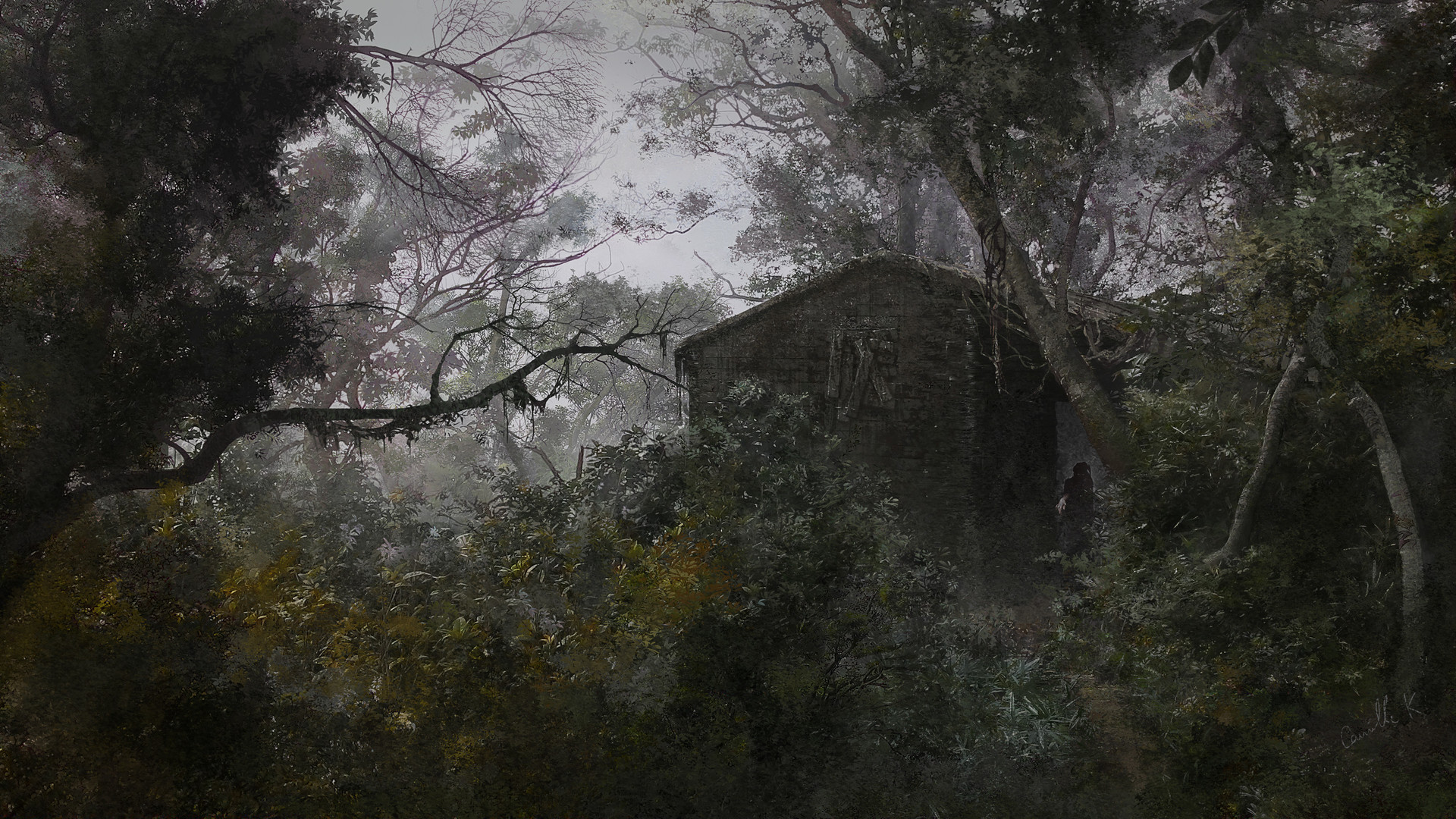The image resembles a painting more than a photograph, exuding a mysterious and eerie atmosphere with its dark, muted, and predominantly gray color palette. Dominated by shades of grays, blacks, and dark greens, there are occasional pops of yellow that stand out against the predominant gloom. The scene is set in a foggy, wooded area with shrubs, bushes, and a dense overlay of trees that add to the overgrown feel of the environment. The central focus is an old, almost dilapidated cabin or shack situated slightly to the right of the composition. This structure appears to be falling apart with wooden pieces haphazardly nailed over one window, giving it an abandoned appearance. Adding to the haunting ambiance, there is a silhouette of a person, possibly a woman, either standing in or near the doorway of the cabin. The background is enveloped in a dense fog, creating a sense of enigma and obscuring further details from view.